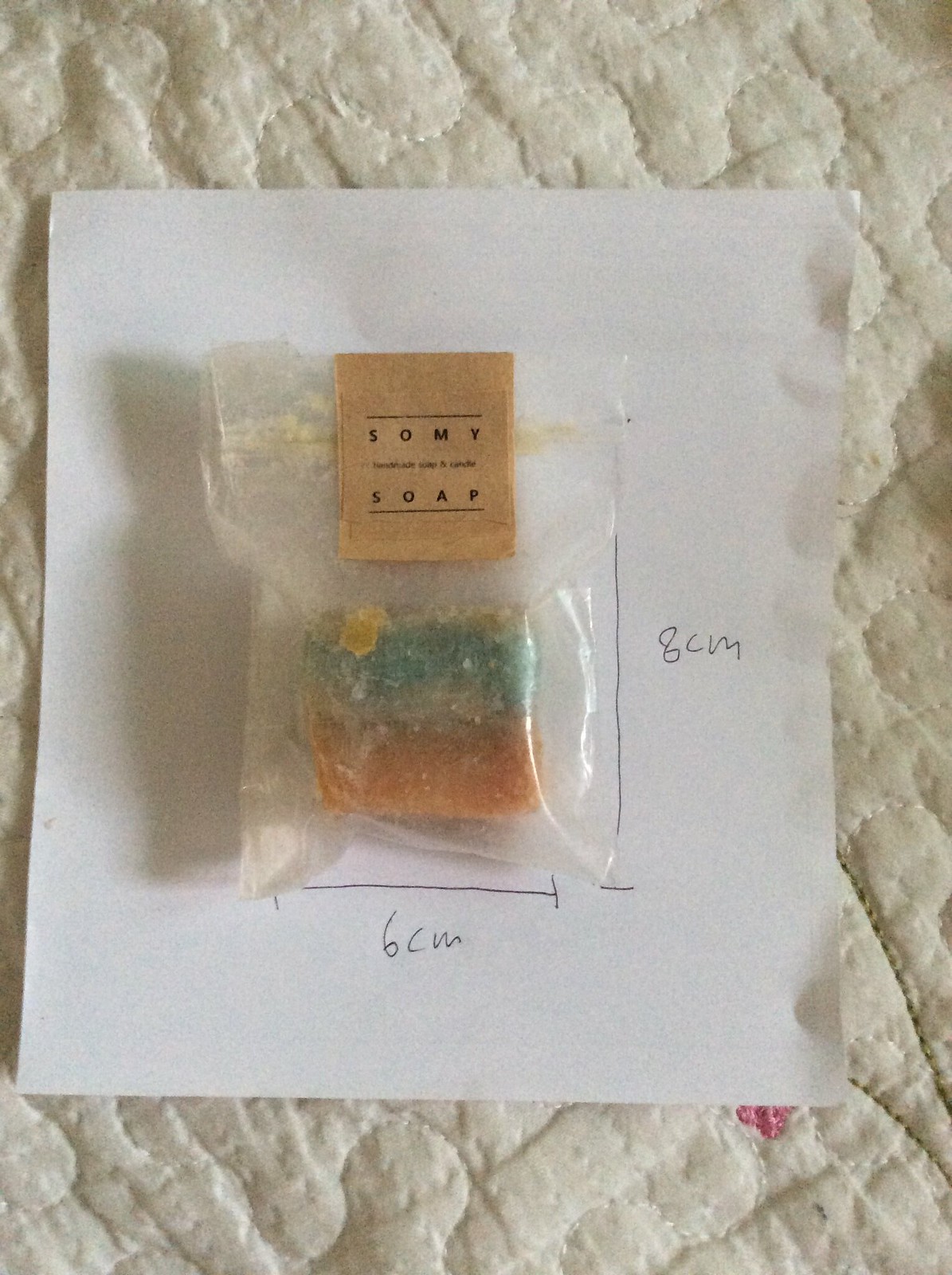In a detailed, close-up photograph, a small, square piece of soap is showcased. The soap, encased in a clear plastic sealed bag, measures approximately 4 centimeters by 4 centimeters and features a distinctive color split: the bottom half is a caramel-orange hue, while the top half is greenish-teal. The bag is affixed with a light brown label at the top that reads "Sew Me Soap" in black text. This setup rests on a white, nearly square piece of paper placed upon a quilted surface, identifiable by the visible patterned fabric around the image's edges. The paper includes hand-drawn measurement lines: a vertical line to the right of the bag indicating a height of 8 centimeters and a horizontal line at the bottom denoting a width of 6 centimeters, giving a clear and detailed context to the dimensions of the soap within its packaging.